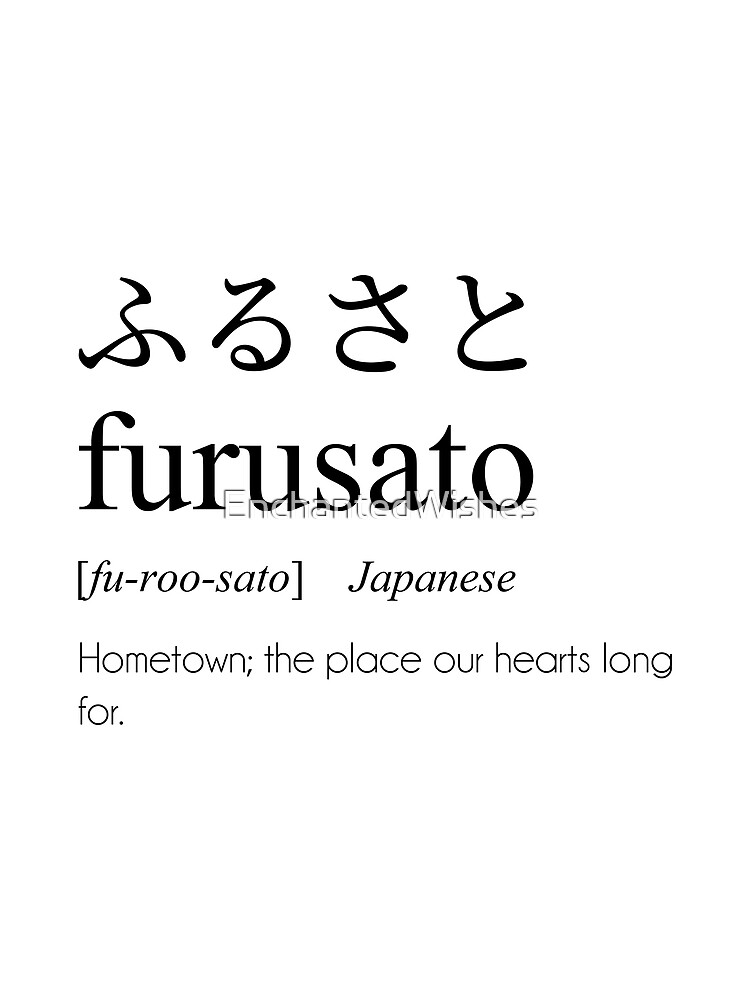The image features a depiction of the Japanese kanji characters for the word "furusato" displayed in an elegant calligraphic style at the top. Below these four black calligraphic symbols, "FURUSATO" is written in large, bold, black serif font. Beneath that, the word "Japanese" appears in italics, accompanied by the phonetic pronunciation "(F-U-R-O-O-S-A-T-O)". At the bottom, in smaller sans serif text, the definition reads: "Hometown; the place our hearts long for." This text is all set against a simple white background and framed by a larger black background. Additionally, a small logo text "Enchanted Wishes" is superimposed over the image. The overall design evokes a feeling of nostalgia and a deep connection to one's place of origin.